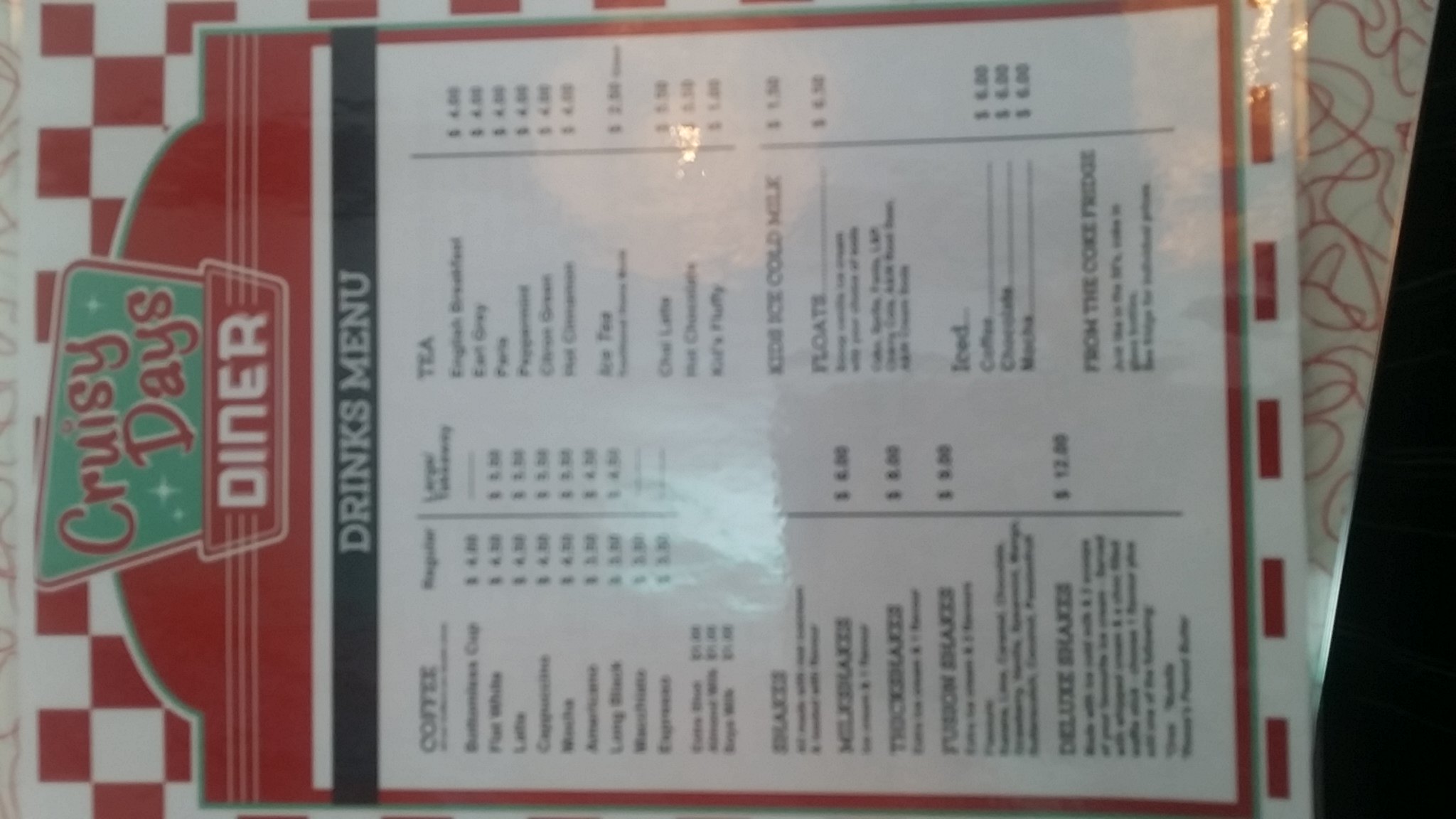This image features a menu resting on a classic 1950s-style countertop, easily identifiable by its white Formica surface adorned with gold squiggly lines. The menu itself isn't upright but instead lies on its left side, requiring viewers to tilt their heads to the left to read its contents. Dominated by red and white colors, the menu sports a nostalgic red-and-white checkered pattern at the top, reminiscent of vintage diners.

At the top center, the text "Cruisy Days Diner" is prominently displayed. "Cruisy Days" is set against a green background with red font, while "Diner" appears on a red background with white font. This is specifically the drinks menu, presented in two columns. The left column lists various types of coffee, while the right column features tea, floats, and additional beverage options that are difficult to discern from the image. The text on the menu is black on a white background, with some drink items accompanied by prices, although these are not legible in the captured photograph.

Additionally, the menu is encased in plastic, evident from the glare of an overhead light bouncing off its surface, adding to the retro ambiance of the scene.